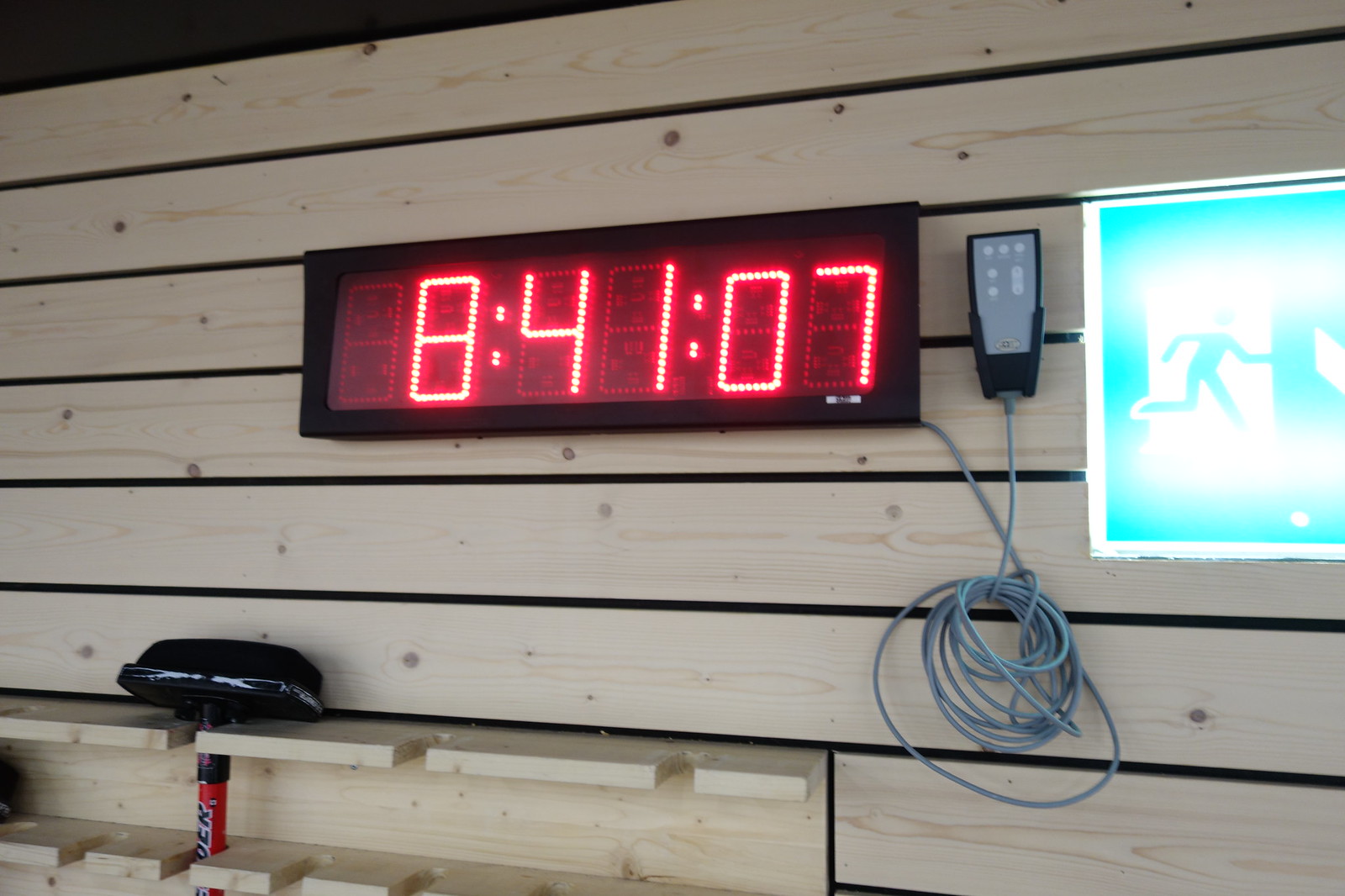In this photo, a digital wall clock is prominently displayed, set against a black face and a red background that strikingly highlights its features. The clock's bright, illuminated numbers display the time as 8:41 and 7 seconds. Adjacent to the clock appears to be a device resembling a phone, likely a remote control for the timer. This entire setup is mounted on a wooden wall, adding a rustic texture that contrasts with the modern electronic components.